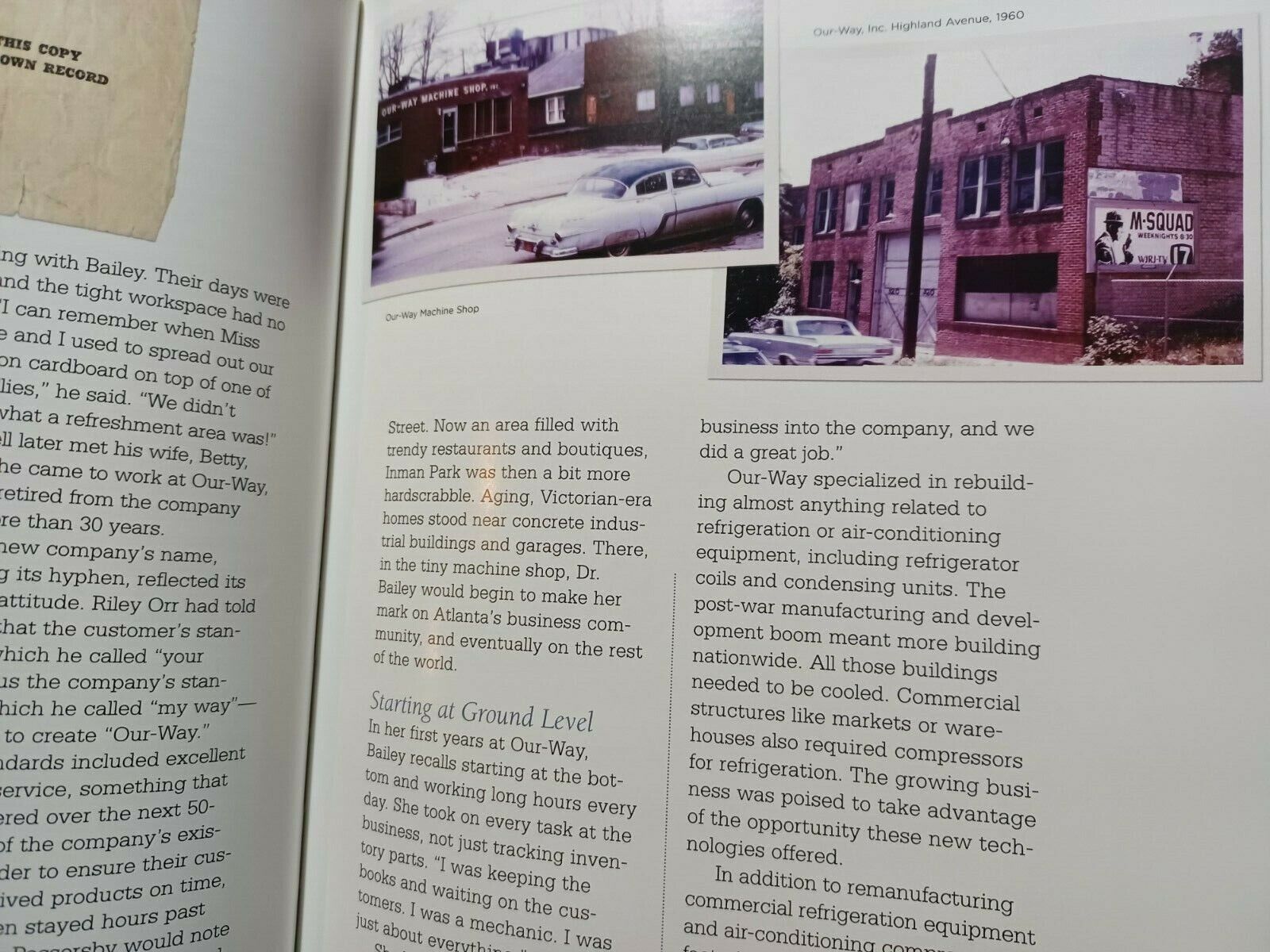The image depicts an open book or magazine, displaying two pages with emphasis on the right-hand page. The right page features two historical photographs at the top, both captioned. The first photo, labeled "Our Way, Inc., Highland Avenue, 1960," shows a building with a car in front of it, suggesting an old, possibly abandoned establishment. The second photo, identified as "Our Way, Machine Shop," portrays a brick building. Below these images, there is text explaining the history of "Our Way" business, detailing its origins in the area of town that specialized in rebuilding refrigeration and air conditioning equipment. The colors in the photos include white, black, deep brick red, gray, and silver, indicating that the images were taken during the daytime. The book or magazine appears to document the business's beginnings and its early environment.